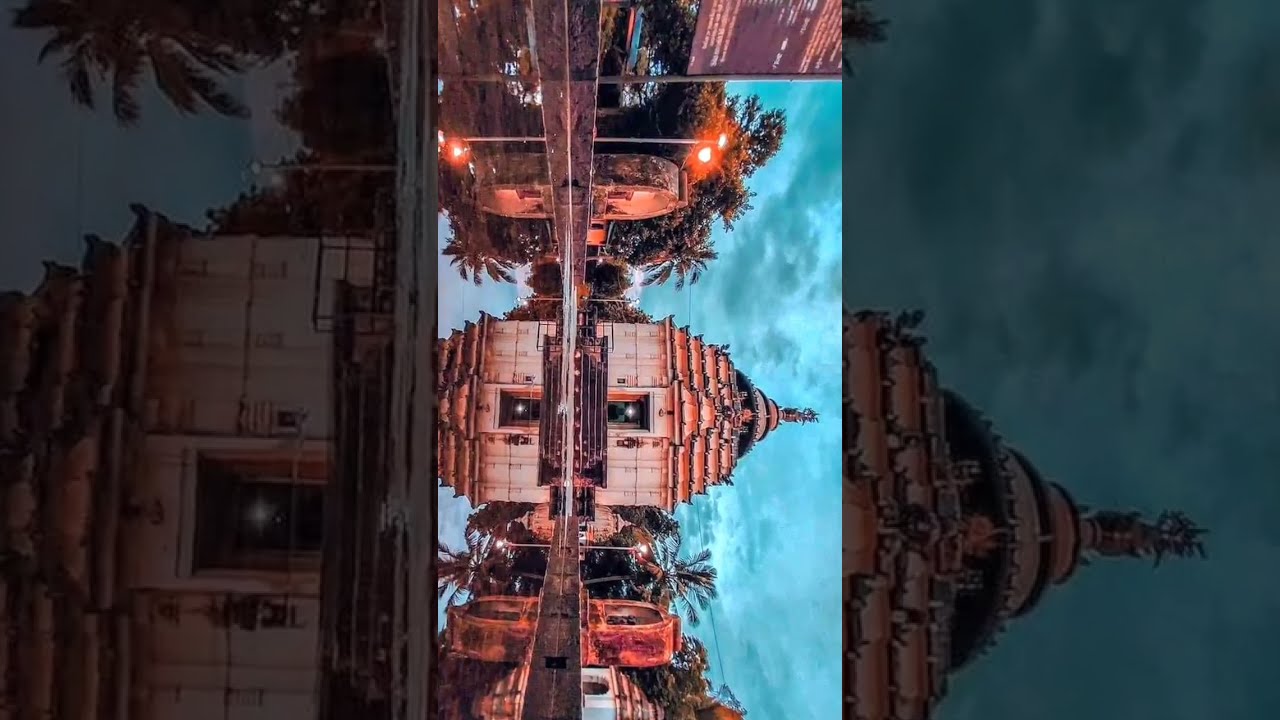This image, captured in extremely high resolution, features an exquisitely ornate stone building with a peach or brown hue. The building's intricate rooftop architecture, composed of several increasingly smaller layers, culminates in a dome-like structure topped with a spire. The picture is rotated 90 degrees to the right, placing the building on its side. The background reveals a strikingly blue, cloudy sky to the right, while a still, mirror-like pool of water lies in front of the building on the left, perfectly reflecting its grandeur.

This outdoor scene is complemented by tall palm trees and smaller structures flanking the central edifice. Streetlights and stone decorative elements can be observed on either side, adding to the picture's detailed beauty. Additionally, a sign is visible to the far left. Enlarged, slightly grayed-out elements of the main image form a calming border, ensuring the viewer's focus remains on the central ornate building and its serene reflection. The light in the image shines from the left, casting gentle illumination over this scene, which seems evocative of a majestic temple or palatial structure.